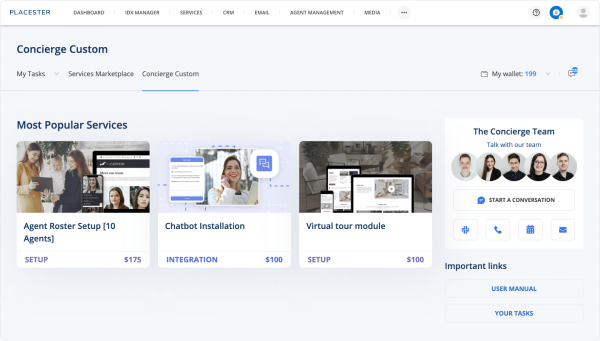The image depicts a small, blurry web page with the header "Playster" in the top left corner. The header features several clickable options including Dashboard, Manager Services, Email, Agent Management, Notification Box, and a Generic Profile Picture. The left sidebar includes navigation items such as Concierge Custom (highlighted with a blue underline), My Tasks, Drop Down Menu, Services Marketplace, and Concierge Custom again. Below the sidebar, a section titled "Most Popular Services" is visible, showing several individuals engaging with what appears to be a tablet or similar device. The following section provides details on services: "Agent Roster Setup," listing 10 Agents with a setup fee of $175.00, and "Chatbot Installation," with integration services priced at $100.00.